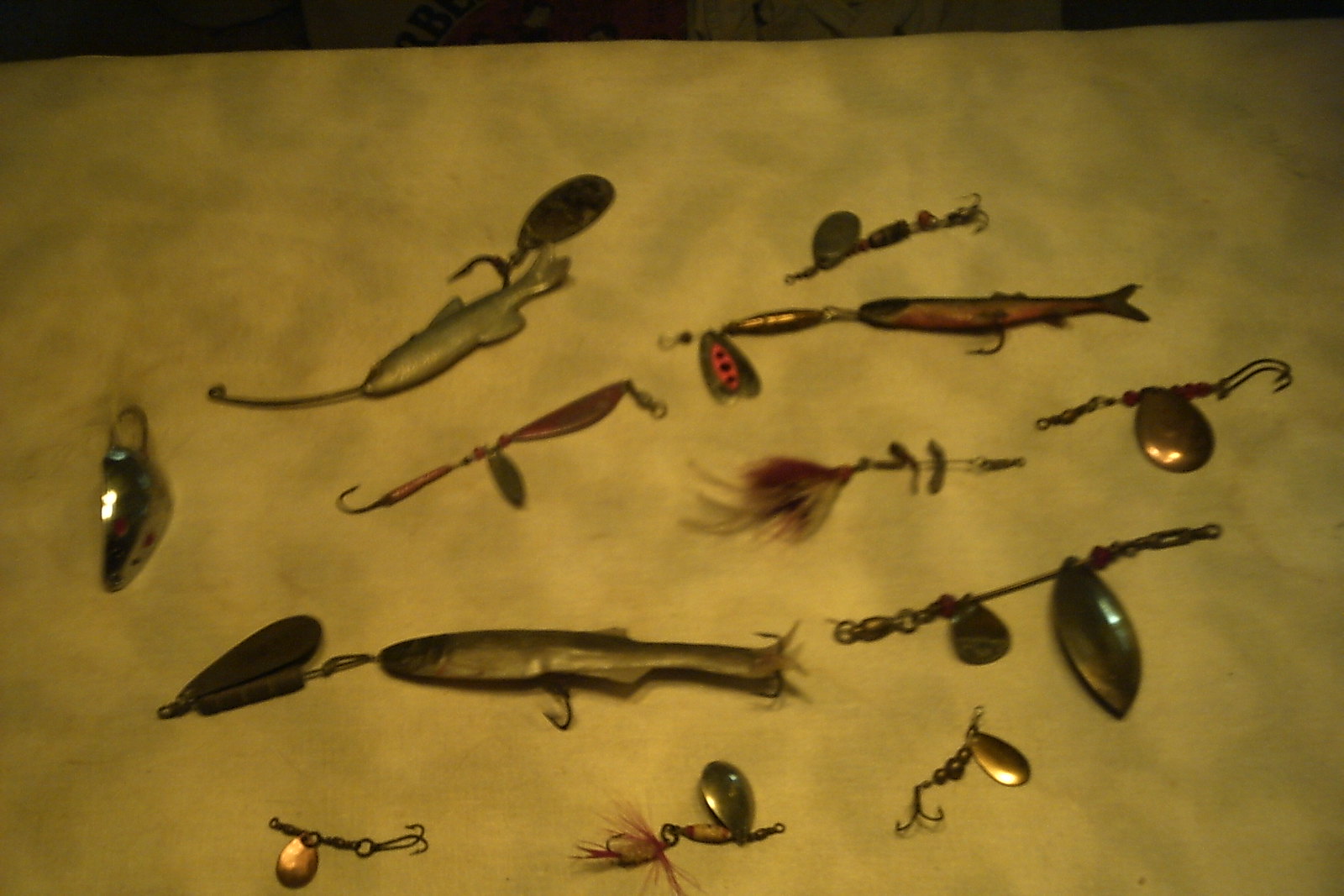This image captures an assortment of approximately 13 fishing lures and tackles, strategically arranged on a flat surface. Each lure is unique, differing in shape, color, and size. Many lures are equipped with metal hooks, some featuring a single curved hook, while others have double hooks. Due to the slightly out-of-focus and low-resolution quality of the photograph, finer details such as the eye patterns on fish-shaped lures are not discernible. The lures include reflective metal and pearl-like elements, and a few are adorned with fur-like strands, possibly to imitate flies. The collection contains varieties such as fly fishing lures and those resembling smaller fish or minnows. The backdrop appears to be a mustard yellow surface with grey marbling effects, further tinted with a greenish-yellow hue due to the overall color tone of the image.